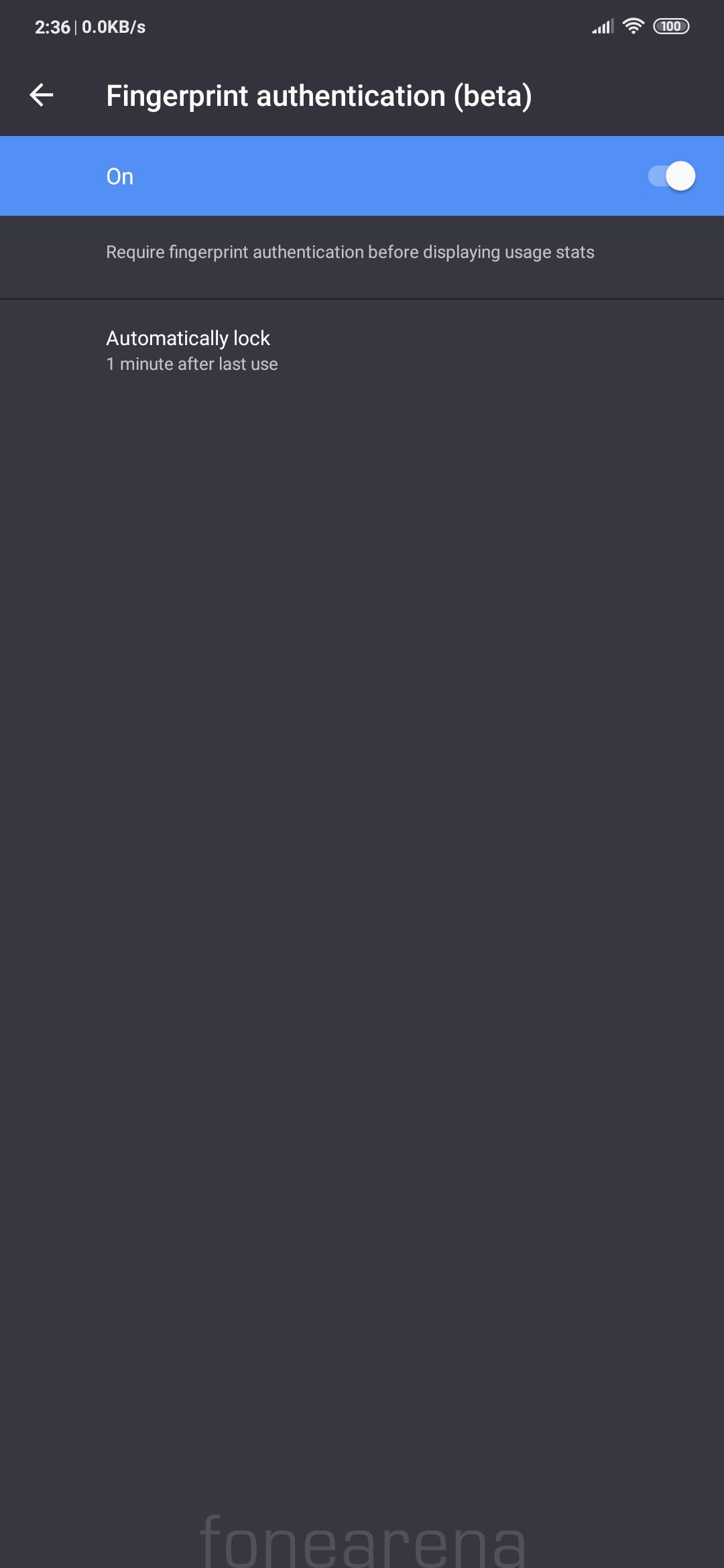This screenshot appears to be from an Android device, distinguished by a "FONEARENA" watermark at the bottom, indicating the source of the image. The device is displaying a time of 2:36, though it is unclear if this is AM or PM. At the top right corner, the status icons reveal that cellular data and Wi-Fi are enabled, and the battery is fully charged at 100%.

Prominently featured in the image is a settings page with 'Fingerprint Authentication (Beta)' toggled on. This setting requires fingerprint authentication before displaying usage statistics. Additionally, the device is configured to automatically lock one minute after the last use.

The background of the screen is a dark silver-gray shade, suggesting that the phone may be operating in dark mode. The layout is sleek and user-friendly, with smaller-than-usual text that enhances clarity and organization. A back button in the form of a left-pointing arrow is visible, further indicating navigation elements typical to Android interfaces.